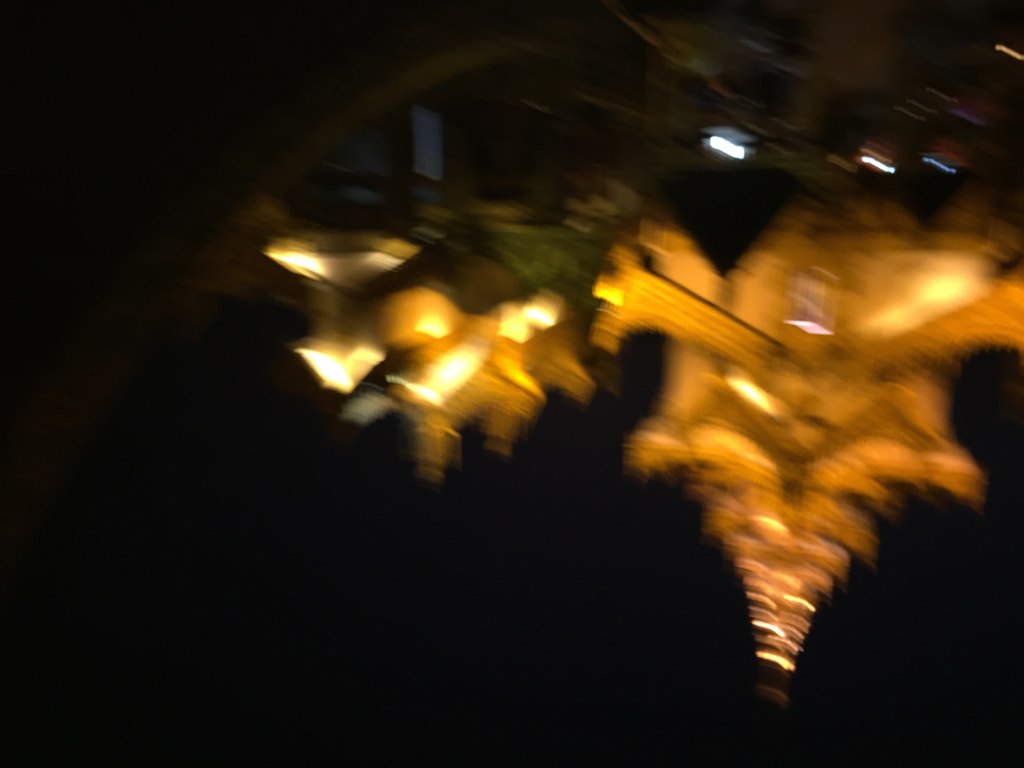This captivating nighttime photograph is characterized by a significant motion blur, transforming the bright yellow-orange light sources into dynamic, flame-like streaks that dance across the composition. The resultant effect infuses the image with a lively sense of motion and energy, although it obscures precise details. The scene likely depicts an urban environment, possibly featuring a street or illuminated architectural structures. The glowing lights may originate from street lamps, windows, or other outdoor illumination sources. The overall impression is one of abstract, chaotic vibrancy, emphasizing the movement of light and color rather than distinct forms. This image evocatively captures the bustling essence of city life after dark.